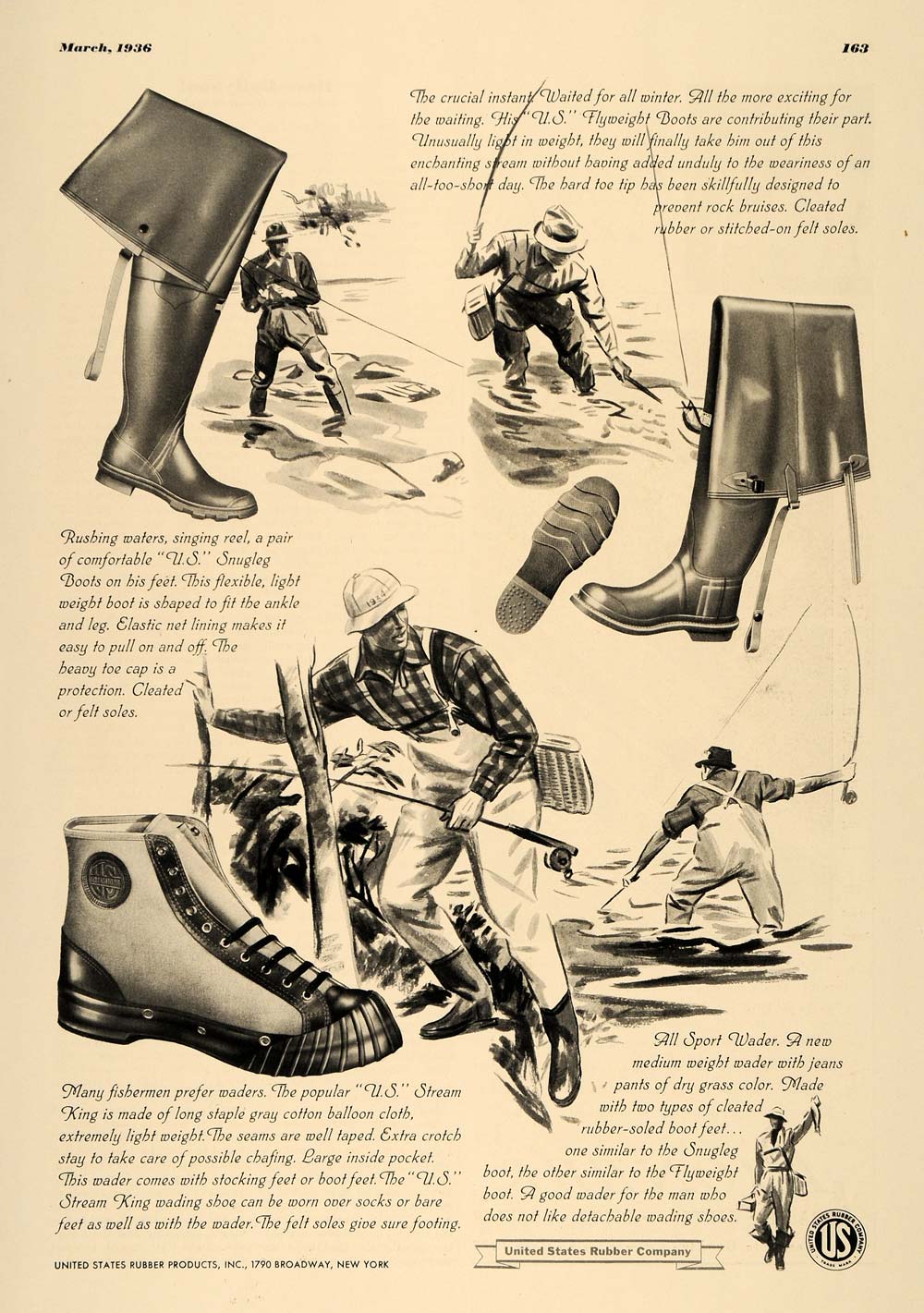This is a vintage full-page advertisement from a March 1936 sporting magazine, showcasing a variety of rubber wading boots for fly fishing. The page, in a beige-tan hue, features "March 1936" in small black letters at the top left corner and "163" at the top right corner. The advertisement displays several detailed illustrations of long thigh-high wading boots, as well as shorter boots, at different angles. Accompanying text describes each boot. In the background, illustrations depict four men engaging in various fishing activities, such as standing knee-deep or thigh-deep in streams, fishing along a lake, or walking by a creek bank. The bottom right corner includes a U.S. logo and an image of a man proudly holding a freshly caught fish.